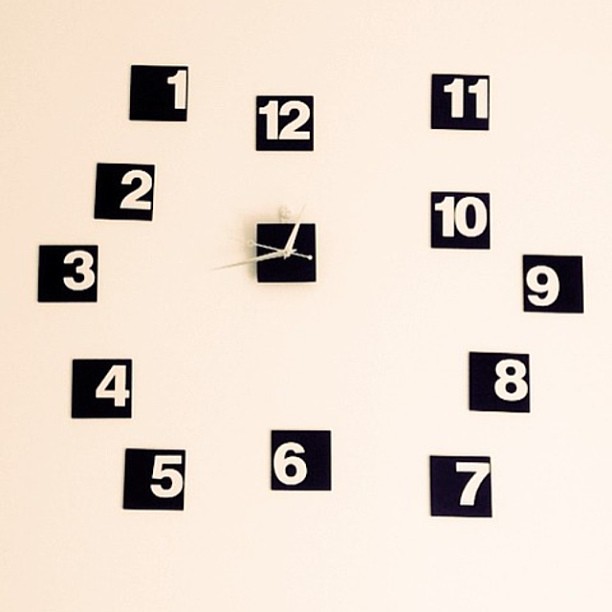The image displays an intriguing and unconventional clock setup against a clean white wall. At the center, there is a minimalistic black square clock, featuring white numbers arranged in an anti-clockwise order around its periphery. The numbers start from 12 at the top, followed by 11 to the immediate right, continuing downwards in reverse sequence: 10, 9, 8, 7, 6, 5, 4, 3, 2, 1. Notably, only the 12 and 6 retain their traditional positions.

This black square clock has two angular gold hands for the hour and minute, which notably extend beyond the edges of the clock’s black square face. Additionally, a second hand is visible, characterized by a filled circle at one end and an open circle at the other, adding to its unique look. The clock indicates the time is approximately 1:40.

The central clock appears to be mounted or hung securely onto the wall and features an additional inner black square, also detailing the clock hands in white. The juxtaposition of the two black squares and the distinctive anti-clockwise arrangement of the numbers provides an artistic and thought-provoking presentation, making this clock a centerpiece within the otherwise plain background.